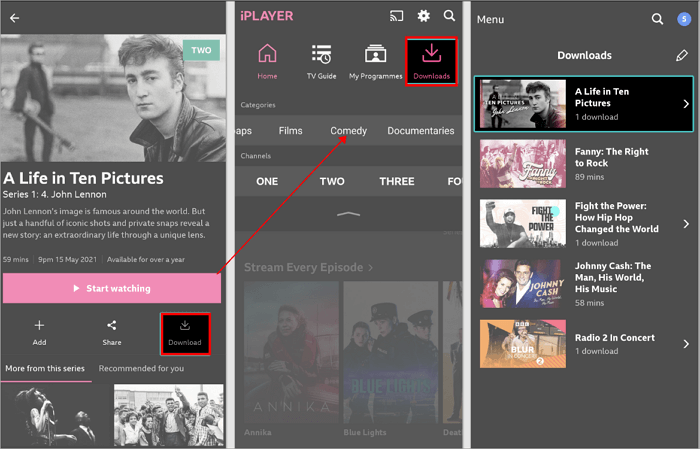This collage comprises three vertical screenshots, likely captured from a mobile device, each showcasing different screens from a streaming service.

In the first screenshot, the black background features a black-and-white image with a small teal banner in the top-right corner displaying the number "2" in white. Below this, the title "A Life in Ten Pictures" appears, indicating it is part of a series. The text beneath reads "Series 1, John Lennon," suggesting this episode focuses on the iconic musician. A summary follows: "John Lennon's image is famous around the world, but just a handful of iconic shots and private snaps reveal a new story—an extraordinary life through a unique lens." Positioned below the description is a pink button labeled "Start Watching." Three icons—"Add," "Share," and "Download"—are displayed underneath, with the "Download" icon marked by a red arrow pointing to the next screenshot.

The second screenshot, titled "iPlayer" at the top, features a trio of smaller icons: "Cast," "Settings," and "Search." Below these, four larger icons are displayed—"Home," "TV Guide," "My Programs," and "Downloads." The "Home" icon is highlighted in pink, while the "Downloads" icon is highlighted in red, aligned with the direction of the red arrow. The screen also presents categories of available series or channels, with the "Downloads" section showing five results: "A Life in Ten Pictures," "Fanny: The Right to Rock," "Fight the Power: How Hip-Hop Changed the World," "Johnny Cash: The Man, His World, His Music," and "Radio 2 in Concert." The first option, "A Life in Ten Pictures: John Lennon," is notably highlighted.

This detailed collage effectively previews a docuseries episode featuring John Lennon, offering options to start watching or manage downloads on the streaming platform.